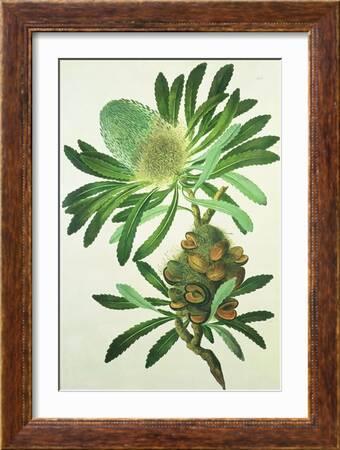This is a framed and matted illustration, displayed against a white wall. The frame is made of medium brown wood, with subtle darker brown streaks adding a touch of design complexity. Inside the frame, a white mat surrounds the artwork, enhancing its presentation with a clean, sharp look.

The illustration itself is an intriguing depiction of a fantastical plant, possibly imagined. The plant features vibrant green leaves and unique, mysterious details. The central element is a bud with several small, open mouths, appearing as though they are seeking something to bite. Above this, another branch extends upward, supporting a cluster of leaves surrounding a bud without the mouths. The leaves are a spectrum of greens, with hints of lighter green and yellow tones.

Adding to the plant's otherworldly appearance, the lower section features what seems like a pale green and cork-colored fuzzy acorn or mossy ball with open clam shell-like structures around it. The detailed artwork, with its blend of natural and fantastical elements, evokes a sense of curiosity and enchantment, making it suitable for display in a museum or a curated store setting.